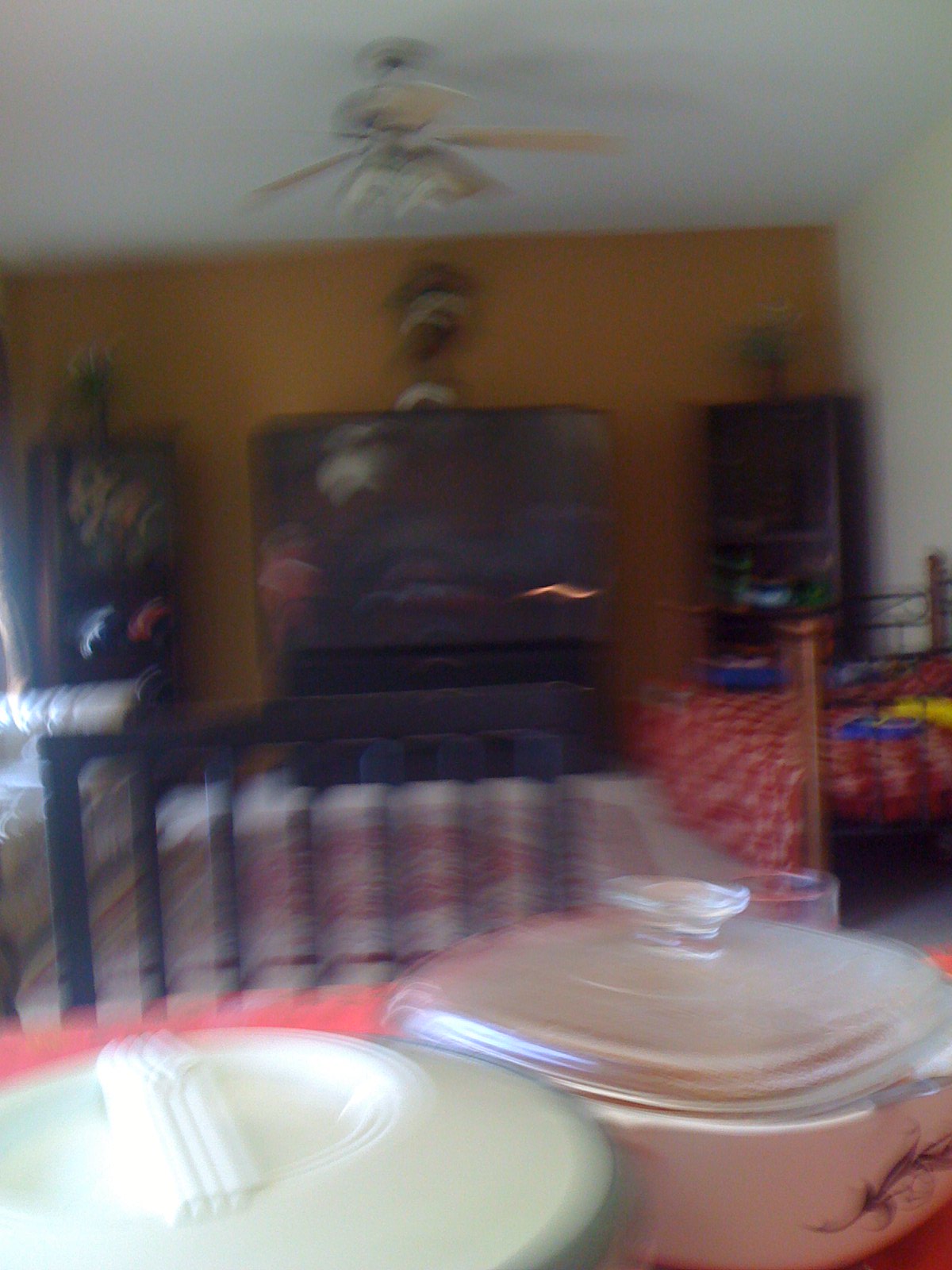This image depicts a rather blurry rectangular portrait taken inside what appears to be a small apartment or home. The foreground features a table, likely a kitchen or dining table, with a red surface barely visible beneath two dishes. On the right side of the table rests a casserole dish that is more square than rectangular with rounded edges. This dish has a glass, slightly domed Pyrex-like lid with a handle on top and a decorative brown leaf-like pattern along the edge. To the left of the casserole dish, in the lower left corner of the image, is a circular plastic container with a nearly white lid and handle that resembles a salad spinner.

The table occupies the bottom quarter of the image. Behind the table is a dark brown wooden chair with an open back, featuring seven vertical bars and a horizontal bar across the top. Only the top of the chair is visible. The background showcases a mustard yellow-brown wall with a large, blurry TV set against it, possibly resting on some furniture. To the right middle of the image is what looks like a low bed with a dark red and white comforter and a brown post at the front, more bed than sofa in appearance.

Further to the back right and back left corners of the room, there are bookshelves. Light filters in from the left side of the room. The ceiling and the right wall are painted white, contrasting with the mustard color of the back wall. A small ceiling fan is mounted on the ceiling. Despite the blurriness of the image, these details provide a glimpse into a cozy, albeit compact, living space.